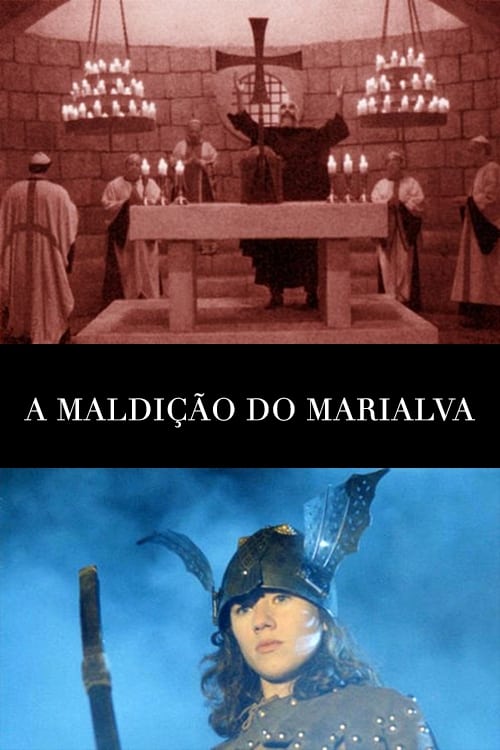The image is a vertically oriented poster, divided into two distinct scenes by a black bar in the center featuring non-English text that reads "A. Maldical du Marlova." The top half of the image has an antique feel, with muted tones of red and shades of brown, white, black, blue, olive, and tan. It depicts a chapel-like setting with a curved brick wall in the background. A group of robed individuals stands in front of an altar, adorned with chandeliers holding candles hanging from the ceiling, and a prominent cross above them. One man, dressed entirely in black, raises his arms in praise towards the cross, surrounded by priest-like figures in prayer. 

In contrast, the bottom half of the poster features a lone figure whose gender is indistinguishable due to their androgynous appearance. This person has shoulder-length, wavy hair and wears full armor, including a Viking-style helmet adorned with bat wing-like extensions. They are holding a sword and a wooden staff. The colors and objects in this scene are also somewhat muted but clearly distinct from the top half, contributing to the overall medieval and mystical ambiance of the image. This detailed imagery suggests the content might be a book cover or DVD cover, shared on platforms like Facebook or Twitter.